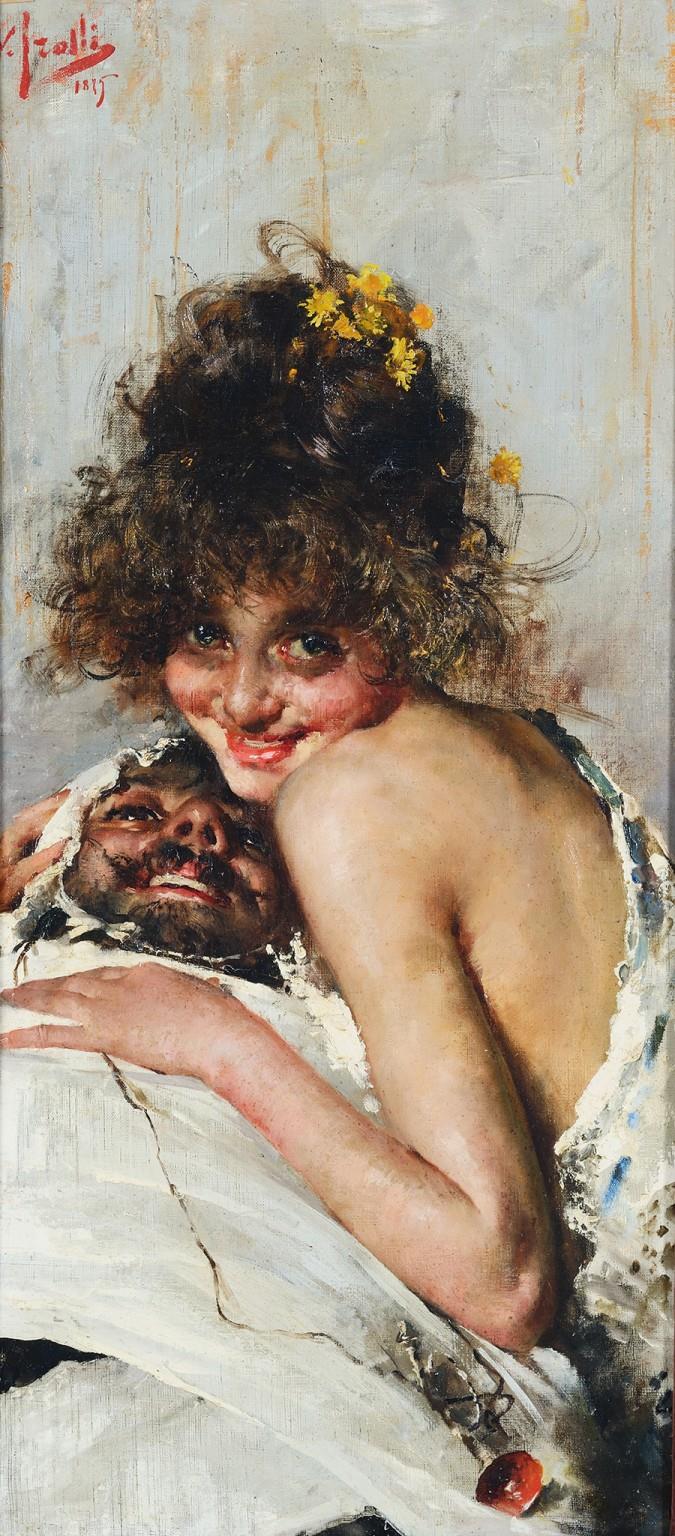This painting, vertical and narrow in composition, features an intimate interaction between a man and a woman who seem deeply connected. The woman, a big-eyed, smiling girl with voluminous dark hair adorned with yellow daisies, is perched beside a reclining man. She is wearing a white dress or skirt that drapes over her right shoulder, leaving her left arm exposed. Her hair, partially up and curly, is held by a floral adornment that adds a touch of whimsy. She gazes directly at the viewer with a radiant grin.

The man, lying down, exudes a contrasting aura of frailty despite his equally warm smile. Sporting a handlebar mustache and beard, he is wrapped in what appears to be a white gown or bandages, with something like a white hat or towel over his head, giving him an almost otherworldly appearance. He holds a small trumpet or horn on a chain, resting on his left hip, adding a curious element to the scene.

Both figures seem to share a profound bond, their expressions suggesting a complex relationship left open to the viewer's interpretation. The artist's signature, a puzzle of letters that begins with "ZULLI," is discreetly placed in the upper left-hand corner, adding a personal touch to this evocative portrait.